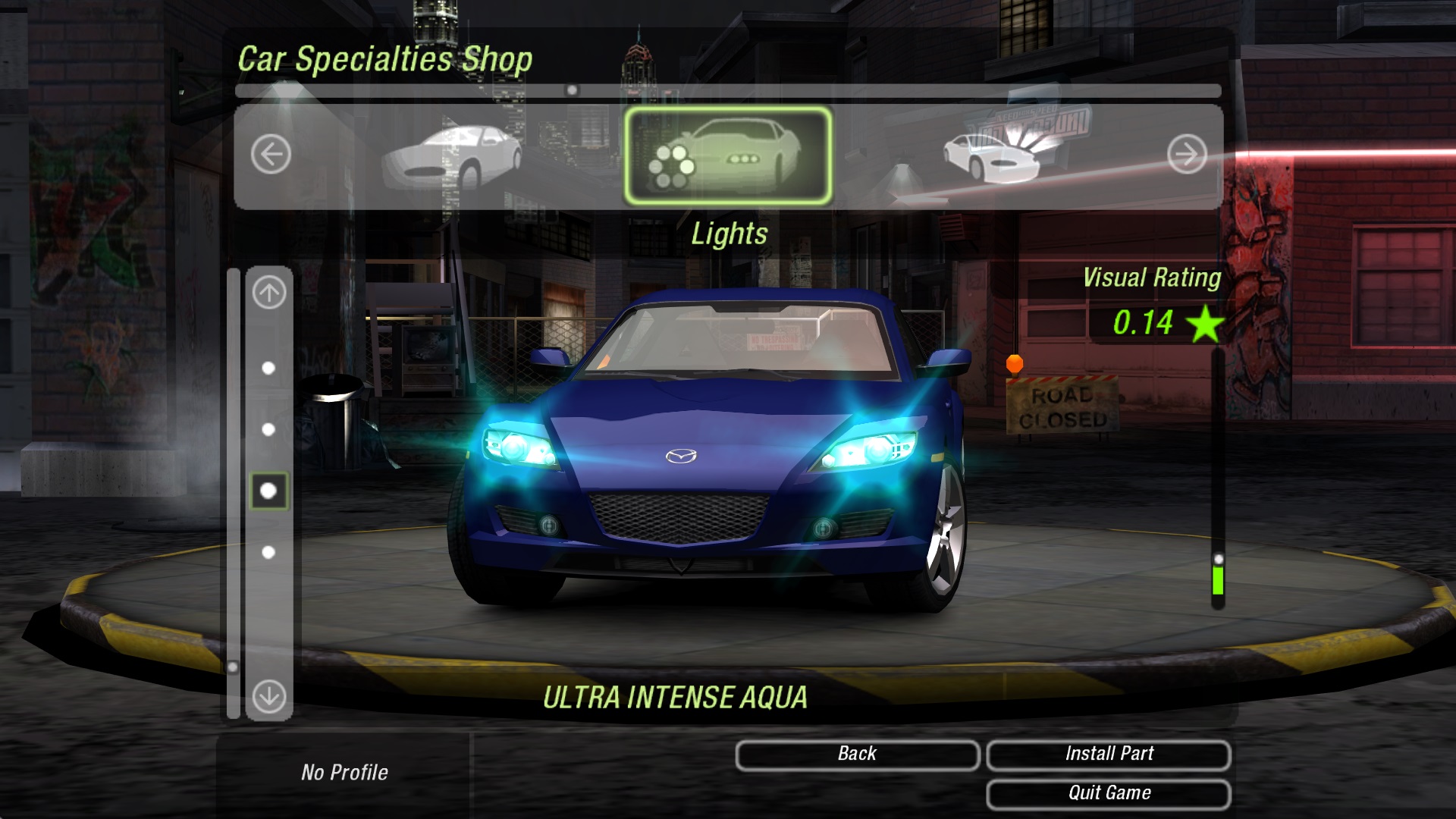This image is a detailed screenshot from a retro video game, likely set in an inner city environment from the PS2 era. Central to the image is a deep blue or electric blue Mazda sedan, possibly mistaken for a Mercedes, with distinct blue headlights, positioned on a spinning disk pedestal. Above this scene, the title "Core Specialty Shop" is prominently displayed in green, suggesting this is a customization menu for the car. The surrounding heads-up display allows players to switch out car parts for performance boosts and aesthetic modifications, featured through menu options and a vertical slider with navigation arrows. The backdrop reveals a dimly lit urban alleyway with graffiti-covered walls, apartment buildings, and closed road signs, adding a gritty, immersive atmosphere to the game’s setting.